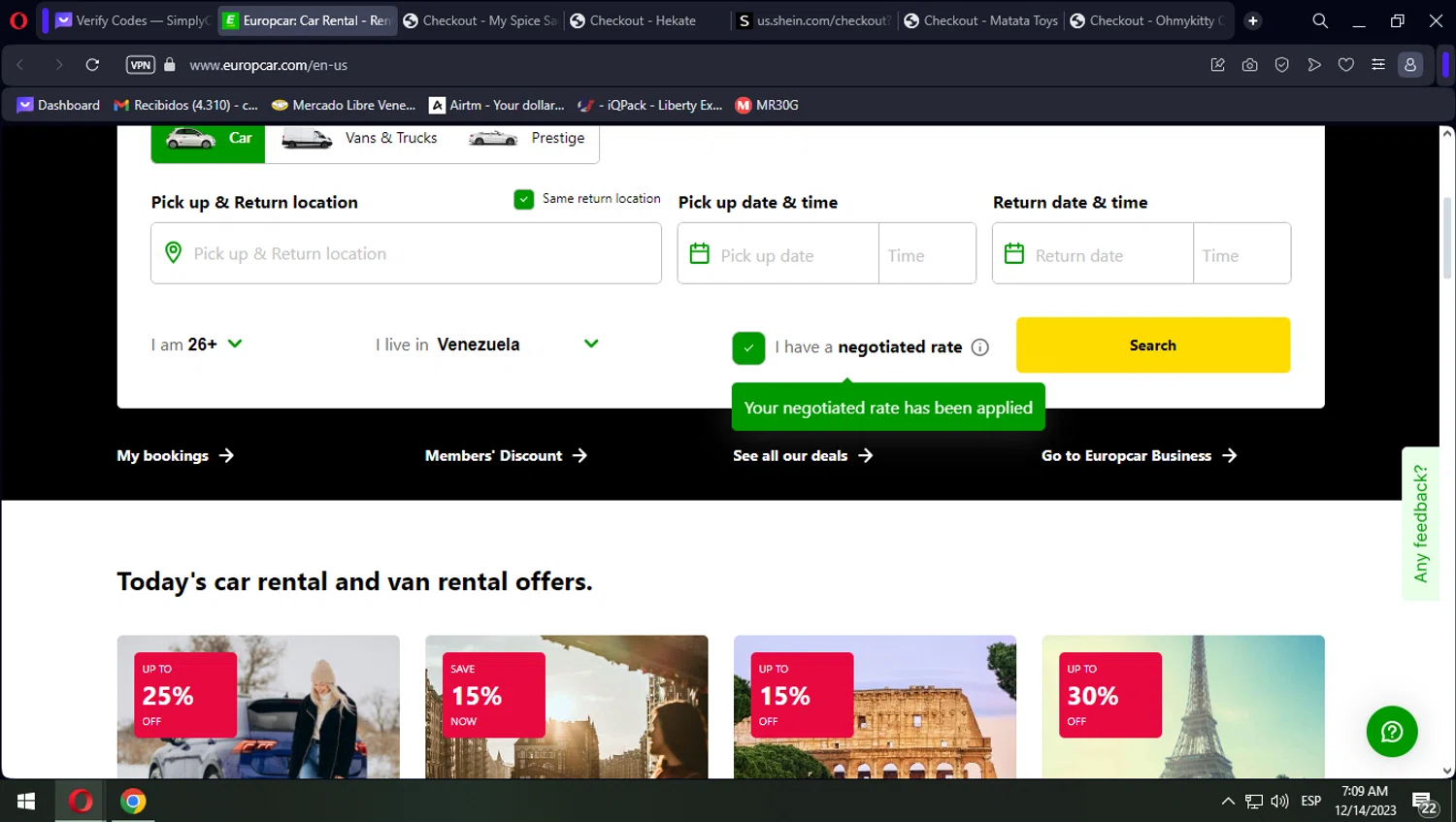The screenshot displays a computer screen with the Opera web browser open, recognizable by the distinctive "O" logo in the top-left corner. Seven tabs are visible, with the one currently active showing the Eurocar Car Rental website. The URL "www.eurocar.com/en-us" is prominently displayed in the browser bar, accompanied by a lock icon indicating a secure HTTPS connection and a label indicating a VPN is active.

The Eurocar Car Rental website homepage offers various options for booking vehicles, including cars, vans, and trucks. Users can proceed by selecting and filling out fields for the pickup and return location, dates, and times. An option is available to toggle if the user is over 26 years old. The site identifies the user's residence as Venezuela, and a checkbox marked in green confirms that a negotiated rate has been applied. A notification below reads "Your negotiated rate has been applied." A prominent "Search" button is nearby for initiating the vehicle search.

Four main categories are listed for navigation:
1. My Bookings
2. Member Discount
3. CR Deals
4. Go to Eurocar Business

Each category is accompanied by a right-pointing arrow. Below this section, headlines promote today's car and van rental offers, positioned under a bold heading "You Save."

The offers are visually presented as follows:
1. An image of a woman with long blonde hair wearing a hat, standing behind a blue car, with a red box overlay that reads "Save up to 25%."
2. A person with long brown hair gazing outside a building, with an overlay box stating "Save 15% now."
3. A picture of the Colosseum in Rome, featuring a box that indicates "Save up to 50% off."
4. An image of the Eiffel Tower, which appears under a partly cloudy sky, with a box offering "Up to 30% off."

At the bottom right of the screen, a green button with a question mark and a talk symbol is available for users needing help or support.